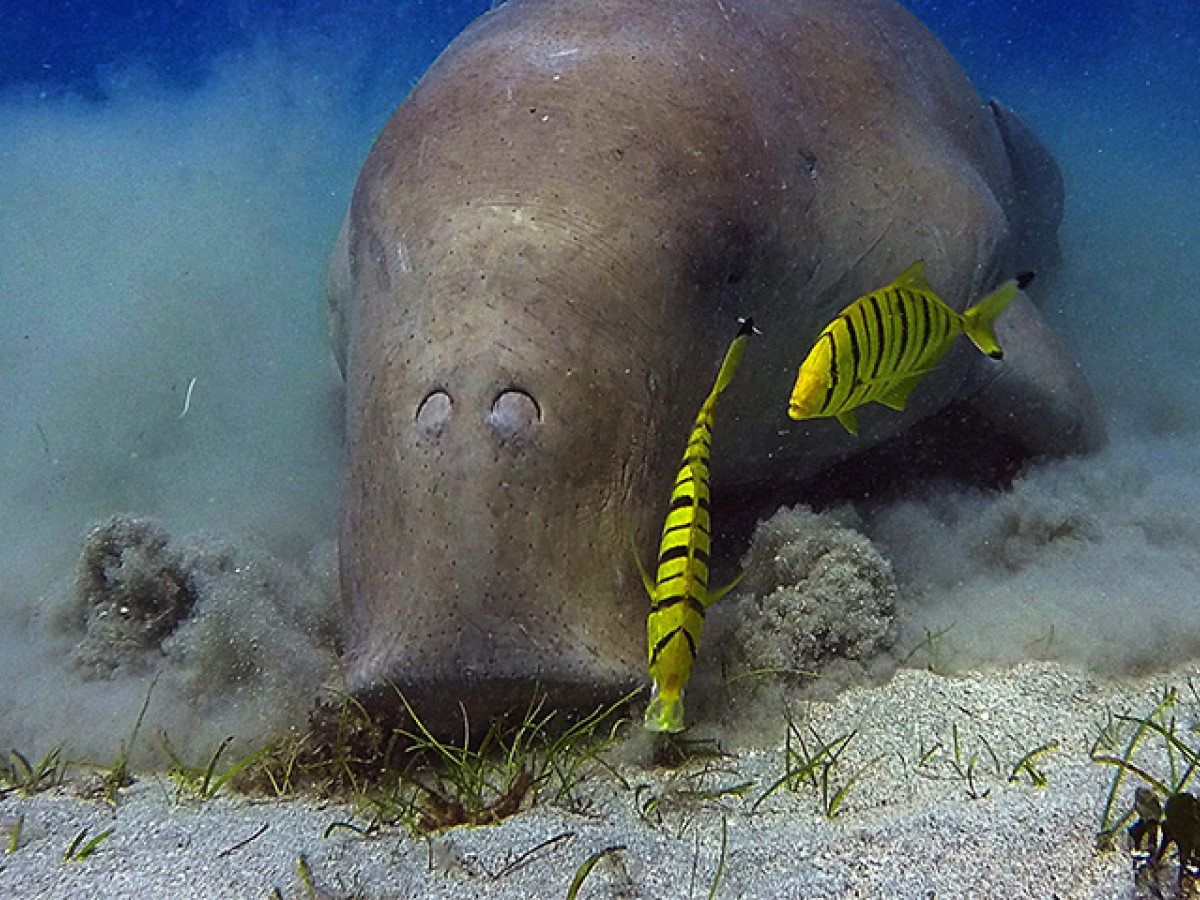This underwater landscape image features a manatee swimming along the bottom of the sea. The photograph captures the manatee from below, with its top portion cut off by the upper edge of the frame. The manatee appears to be sifting through the sand, creating a dusty, cloudy effect as it disturbs the seabed. The sandy bottom is scattered with small pieces of grass and dirt. Surrounding the manatee, the water appears blue, especially noticeable at the top of the image. To the right of the manatee, two large yellow fish with black vertical stripes and black tips on their tails are visible, contrasting sharply with the dusty, disturbed sand. The image is devoid of people and text, focusing solely on the natural underwater scene.